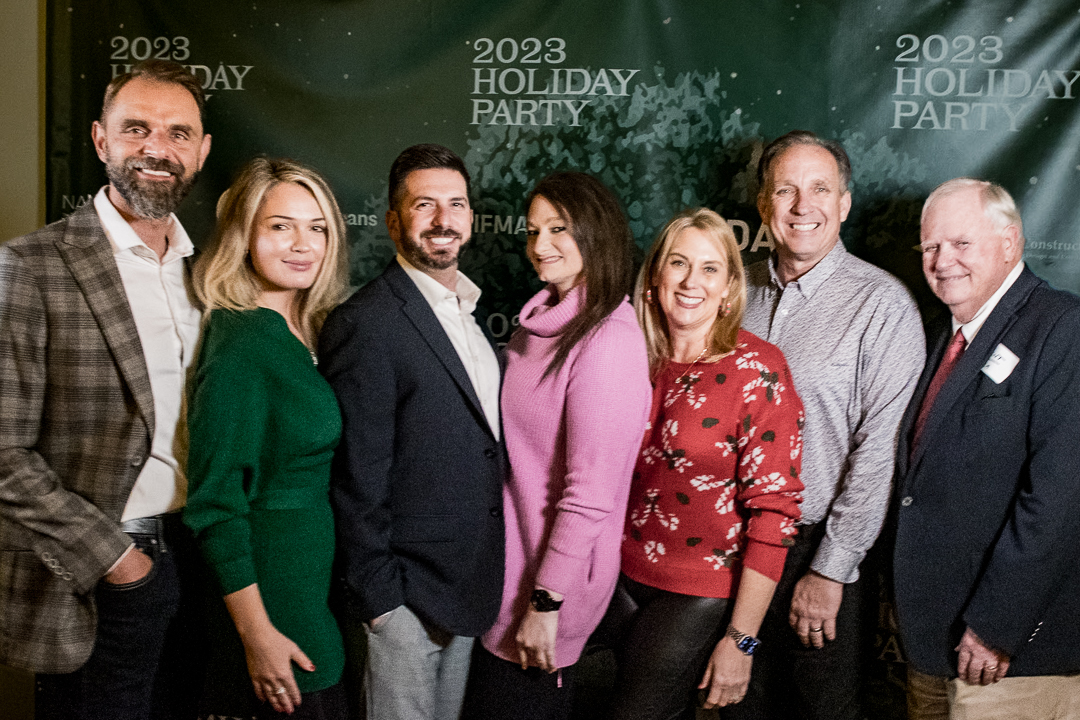This is a detailed photograph capturing a group of seven people, composed of three women and four men, standing aligned next to each other at what appears to be an office or corporate holiday party. They are positioned in front of a wall featuring a green drapery backdrop that prominently displays the phrase "2023 Holiday Party" multiple times. The background also includes a geometric design, a logo, and an image that is partially obscured by the group, which adds to the festive decor with some red dust arranged to look like snow.

The individuals in the photo display a casual, yet professional dress code; the women are dressed in nice sweaters, while the men are in button-down shirts and blazers or suits. Specifically, the man on each end of the line, as well as the second man from the left, are wearing suits, whereas the man positioned before the rightmost individual wears a gray shirt. The scene suggests a relaxed atmosphere symbolizing camaraderie among colleagues celebrating the holiday season together.